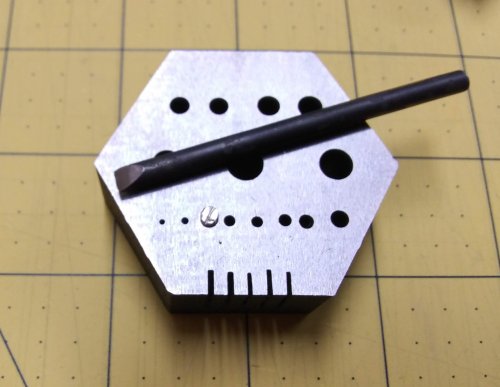In this detailed image, a hexagonal steel bit gauge rests upon a medium brown tile background with a subtle dotted pattern in three rows of three, bordered by black grout. The steel gauge exhibits a structured array of perforations: a top row of four small holes, a middle row of three significantly larger holes, and a bottom row of eight holes that progressively increase in size from left to right. The lower portion of the gauge also features five distinct cut lines. Positioned diagonally across this bit gauge is an iron rod or chisel, characterized by a flattened end that transitions into a rounded shape.